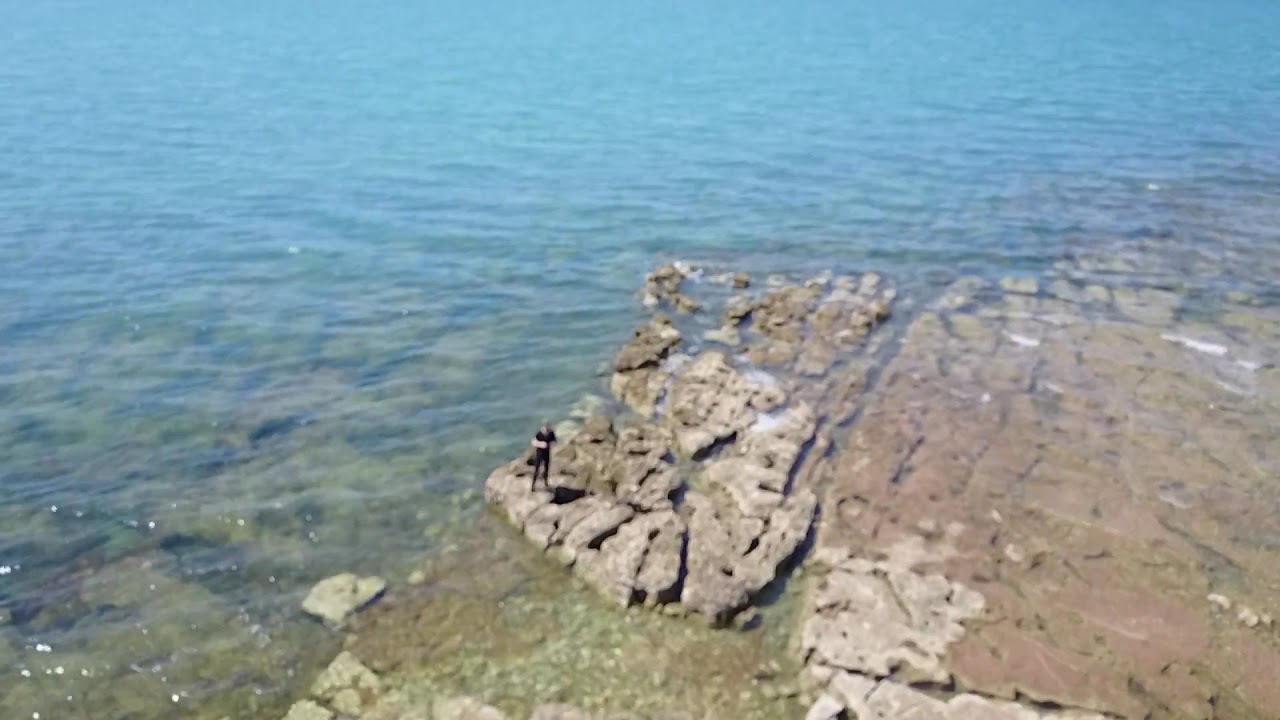The photograph captures a scenic and well-lit body of water, predominantly occupying the middle and upper sections of the image. The water ranges from a pristine, light blue in the upper half to a clearer state in the foreground, revealing an array of stones and rocks beneath the surface. The lower right and middle right portions of the picture feature a rocky area, with larger, craggy, and brown stones emerging from the water. These stones, partially submerged and covered in areas by darker hues, perhaps from algae, contrast with the lighter, dry stones in the center of the image.

In the middle of the scene, a person dressed in black pants and a black shirt stands on these stones. Although they appear small due to the high vantage point of the photograph, akin to a perspective from a cliff, their posture suggests they are looking down at something, possibly the stones or water beneath them. Gentle waves ripple across the water's surface, adding to the serene atmosphere of the bright, sunlit day. The interplay of gray, tan, and blue tones in the rocks and water, along with some indistinct greens, creates a harmonious and picturesque landscape.